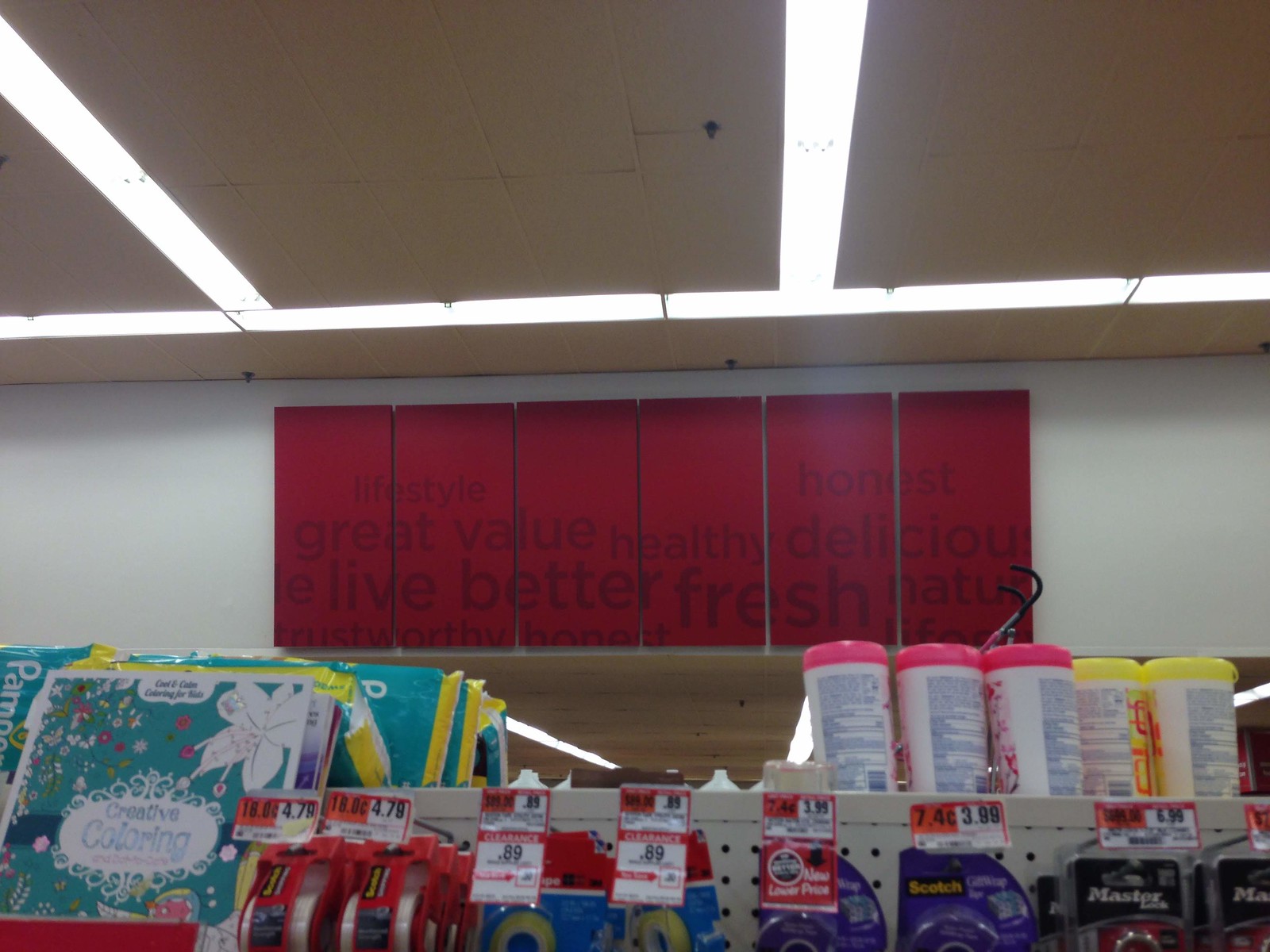The photo, taken inside a bustling shopping center, showcases the rear section of a well-lit store. Dominating the back wall is a series of six contiguous red panels, collectively emblazoned with uplifting and consumer-friendly words such as "lifestyle," "honest," "great value," "health," "delicious," "live better," "fresh," "natural," "trustworthy," and "honest." Below these motivational panels lies a retail shelf neatly arranged with various products. To the right, a prominently displayed Pampers section catches the eye, featuring diapers and a creative coloring book placed in front of them. Adjacent to this, a metal peg shelf is stocked with assorted types of tapes, each tagged with red and white price labels, indicating that two of the items are on clearance. Atop this peg shelf, several containers of wipes are orderly positioned, suggesting convenience and accessibility for shoppers. The detailed arrangement of the store reflects an organized and customer-centric environment.